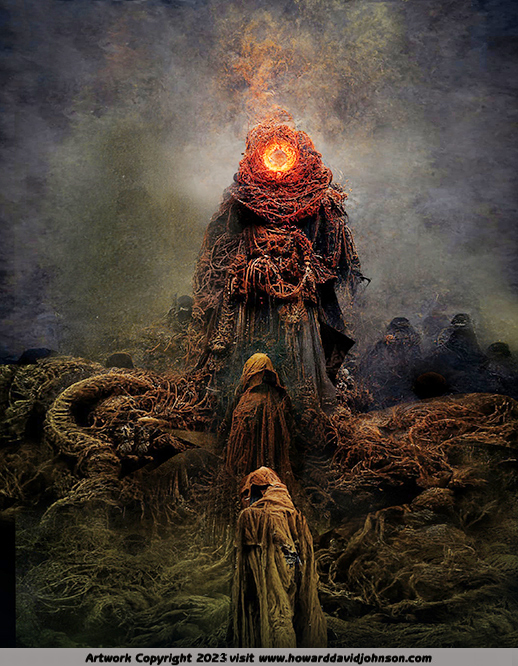This detailed fantasy artwork exudes a dark and eerie atmosphere. At the forefront, we see two hooded figures—one closer to the viewer at the bottom of the image, and another slightly higher up on a small hill—both dressed in tattered, dirty robes. Towering over them in the center of the composition is an immense, ominous figure. This central entity has an unsettling, organic appearance, adorned with what seem to be roots, twines, and red-colored necklaces that dangle from its chest, contributing to its monstrous guise. Its head is not a typical face but a large, glowing orb, yellow with an orange square at its core, emanating plumes of smoke as if on fire. The background is filled with more shadowy, hooded figures, adding to the scene's creepy and surreal nature. The landscape features gnarled roots and snaking vines, reminiscent of HR Giger's biomechanical style, yet with a more organic twist. The sky above is dark, gray, and smoky, further enhancing the menacing and otherworldly mood. A watermark at the bottom of the image reads "artwork copyright 2023. Visit www.howarddavidjohnson.com," indicating the artist's credit.